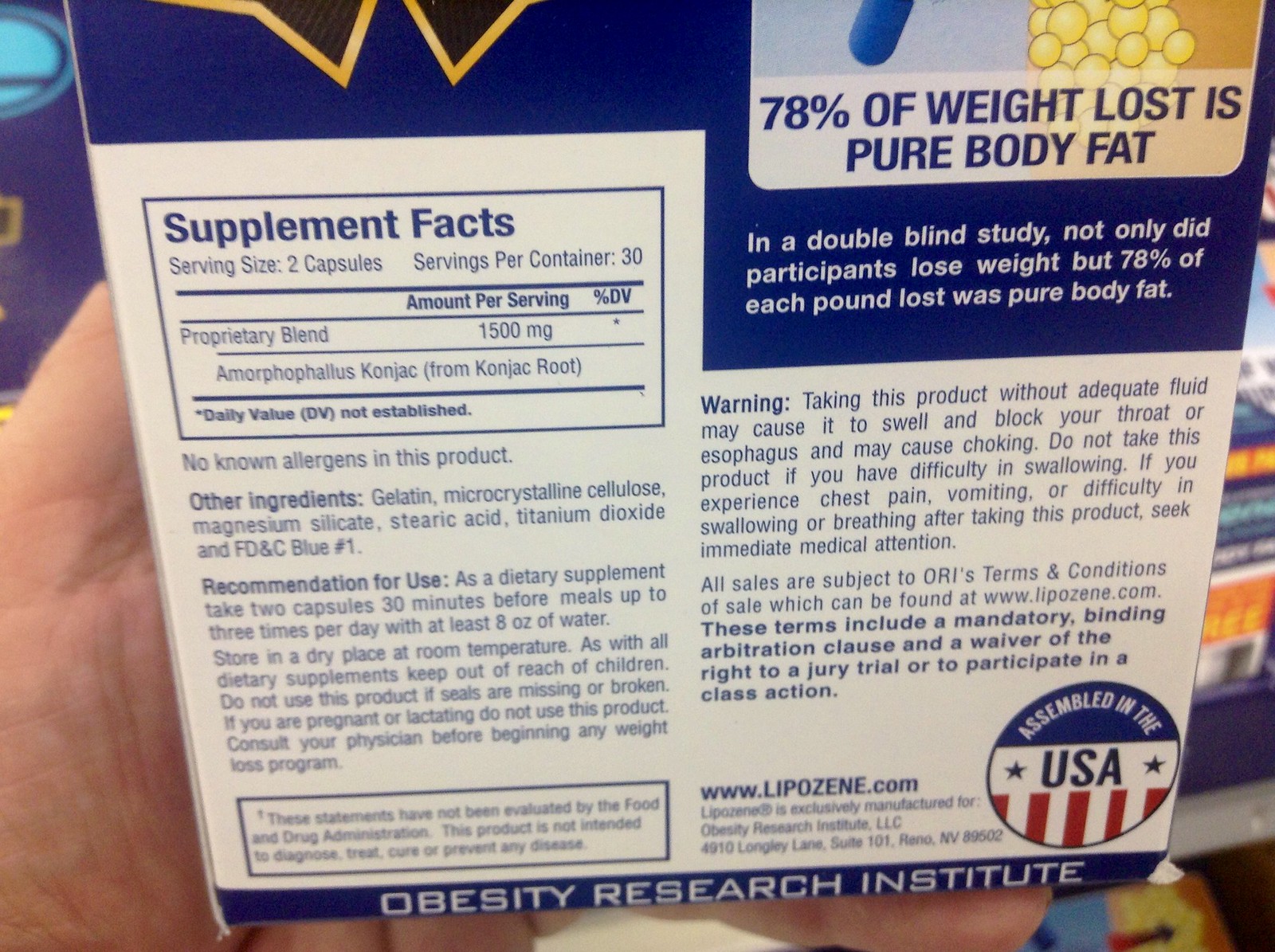This image features the back of a carton for a dietary supplement called Liposene. The carton, held up by a person on the left side of the frame, is predominantly white with a blue section at the top. Highlighted in the top-right corner is the claim "78% of weight lost is pure body fat," and an explanation follows that in a double-blind study, participants' weight loss comprised 78% body fat. Below this, the Supplement Facts section specifies a serving size of two capsules, with each serving containing a proprietary blend of 1,500 milligrams, including konjac root, and assures no known allergens are present. The bottom-right corner features a logo indicating it is assembled in the USA, with red and white stripes at the bottom and a blue upper segment, accompanied by the label of the Obesity Research Institute.